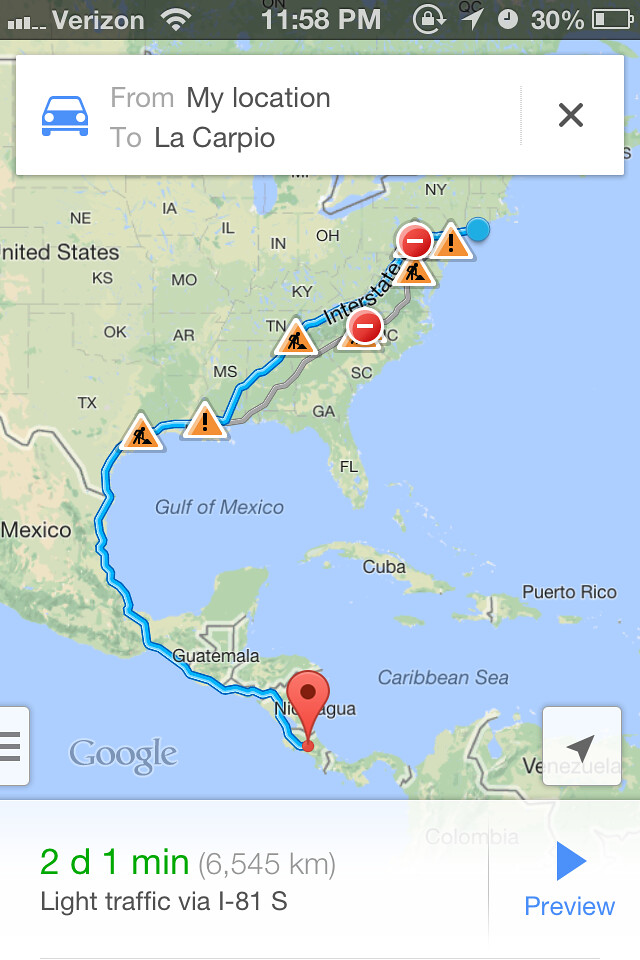A detailed road map screenshot showcases a planned journey from Delaware to an undisclosed location in Costa Rica, prominently displayed on a Google Maps interface. The image is square with a black bar at the top, announcing Verizon as the service provider, with a full-strength signal at 11:58 p.m. The user's battery is at 30%. The current location is indicated with a blue circle. The meticulously plotted route spans the eastern United States and most of Central America, highlighted in blue. The map, covering approximately half ocean, details various construction zones and points of interest along the way, with an alternate route marked in gray. The total journey is estimated to take two days and one minute, covering a distance of 6,545 kilometers, with light traffic reported on I-81 South.